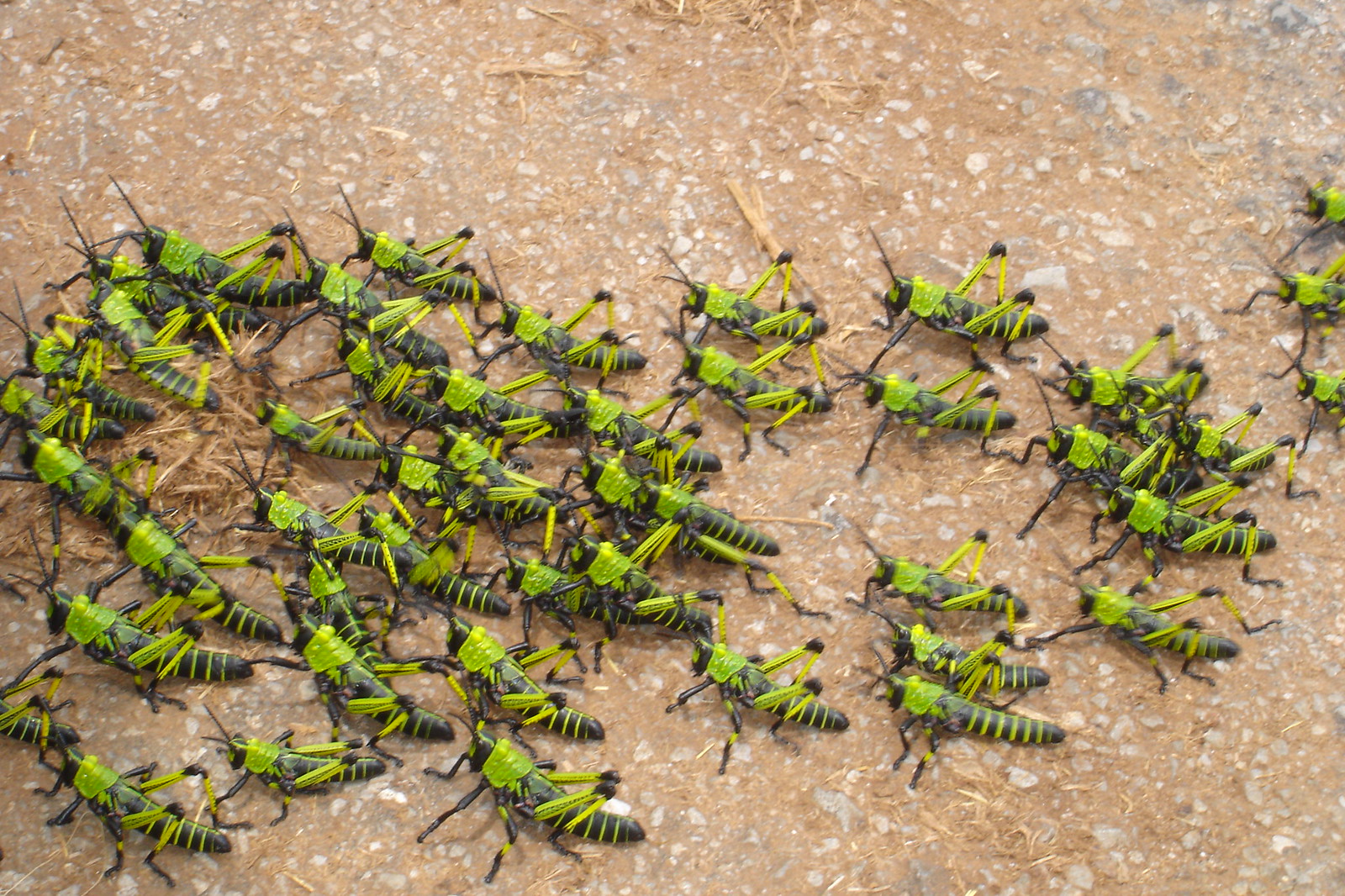The image captures a large assembly of around 30-50 grasshoppers or locusts, noticeable for their striking color pattern of black bodies accented with bright neon green along the thorax, legs, and stripes across their abdomens. Each insect features two black, slender antennas protruding from the top of their heads, which also bear a distinct green spot. They are situated on a reddish-orange gravel path interspersed with white rocks and small brown sticks or wood shavings. The insects predominantly face the left side of the photograph, suggesting a coordinated movement or possibly seeking sunlight. The overall scene is both intriguing due to the vivid colors and unsettling given the sheer number of insects densely packed together on the rugged terrain.